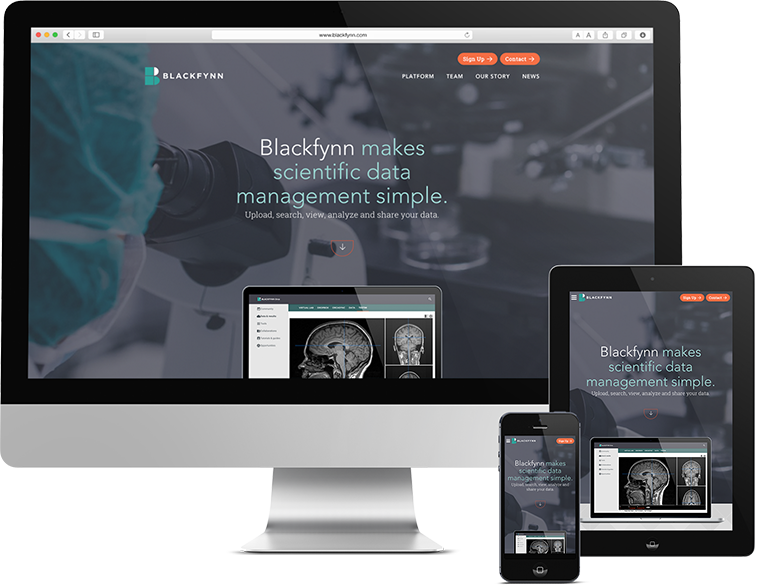This image showcases a web page displayed across multiple devices: a MacBook computer centrally positioned, a tablet at the bottom right, and a smartphone in front of the tablet. All devices depict the same content. 

In the top left corner of the webpage, the word "Blackfin" is prominently featured alongside a green and white bee icon. The top right corner displays two patterned orange buttons labeled "Sign Up" and "Contact." Below them are navigation tabs labeled "Platform," "Team," "Our Story," and "News."

Centrally, the webpage contains a bold message in white and green text: "Blackfin. Make scientific data management simple. Upload, search, view, analyze and share your data." Beneath this message, an image of a laptop screen displays an X-ray of a human skull, highlighting detailed views of the brain and surrounding structures. This visual element emphasizes a scientific theme.

In the background, a person is depicted on the left side of the screen, peering through a black and white microscope. The individual is wearing protective gear, including a blue head cover and a white mask, suggesting a laboratory setting. This detailed composition underlines Blackfin's focus on scientific data management.